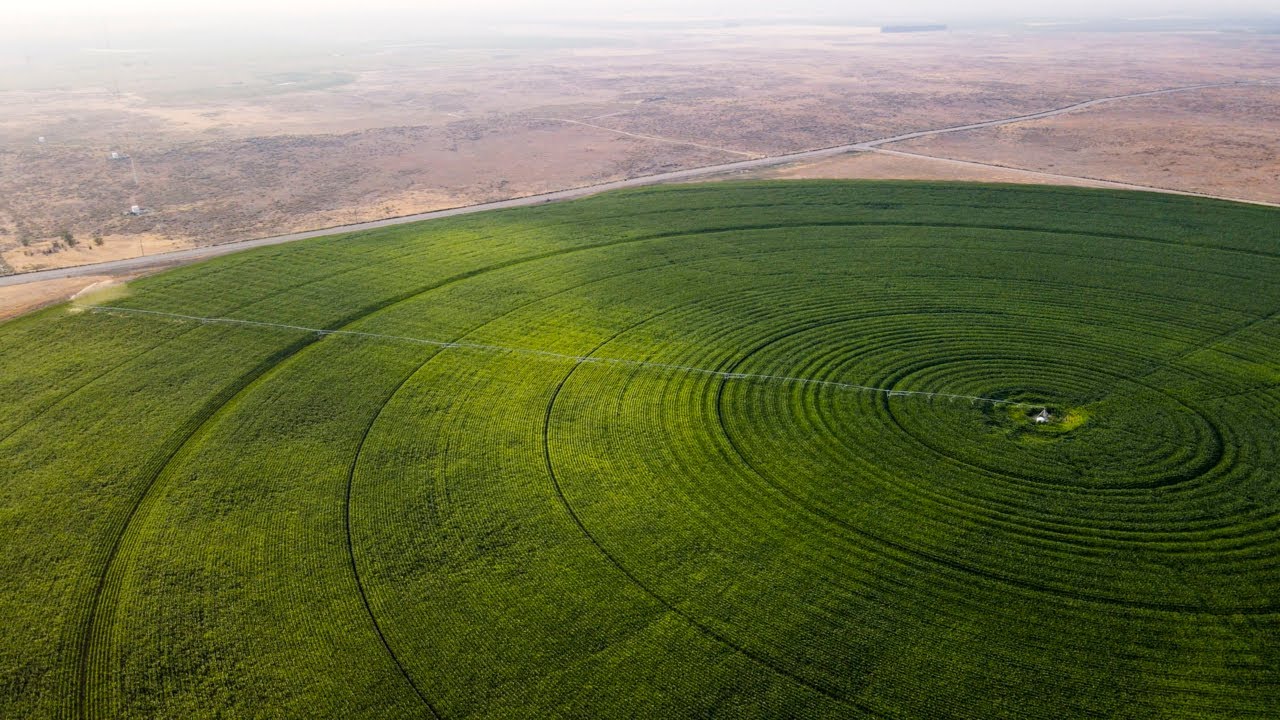A drone-captured image reveals a series of circular cornfields nestled within an arid, desert-like region of Southwest Idaho. The aerial view highlights the vast expanse of green, meticulously irrigated cornfields contrasting starkly with the surrounding barren landscape. These circular fields are an ingenious product of pivot irrigation systems, where long arms rotate around a central pivot, ensuring even water distribution across the fields. This sophisticated irrigation enables the cultivation of corn in an otherwise inhospitable environment. The image features a prominent white section at the center of one of the circles, possibly indicating a control or maintenance hub for the irrigation system. A path, also appearing white, extends from the upper left exterior of the cornfield and traverses into the center. The picturesque scene is framed by the backdrop of the desert, characterized by gray and brown tones, with a road cutting through from the left center to the upper right corner, underscoring the isolation of these lush, man-made agricultural plots amidst the dry expanse.